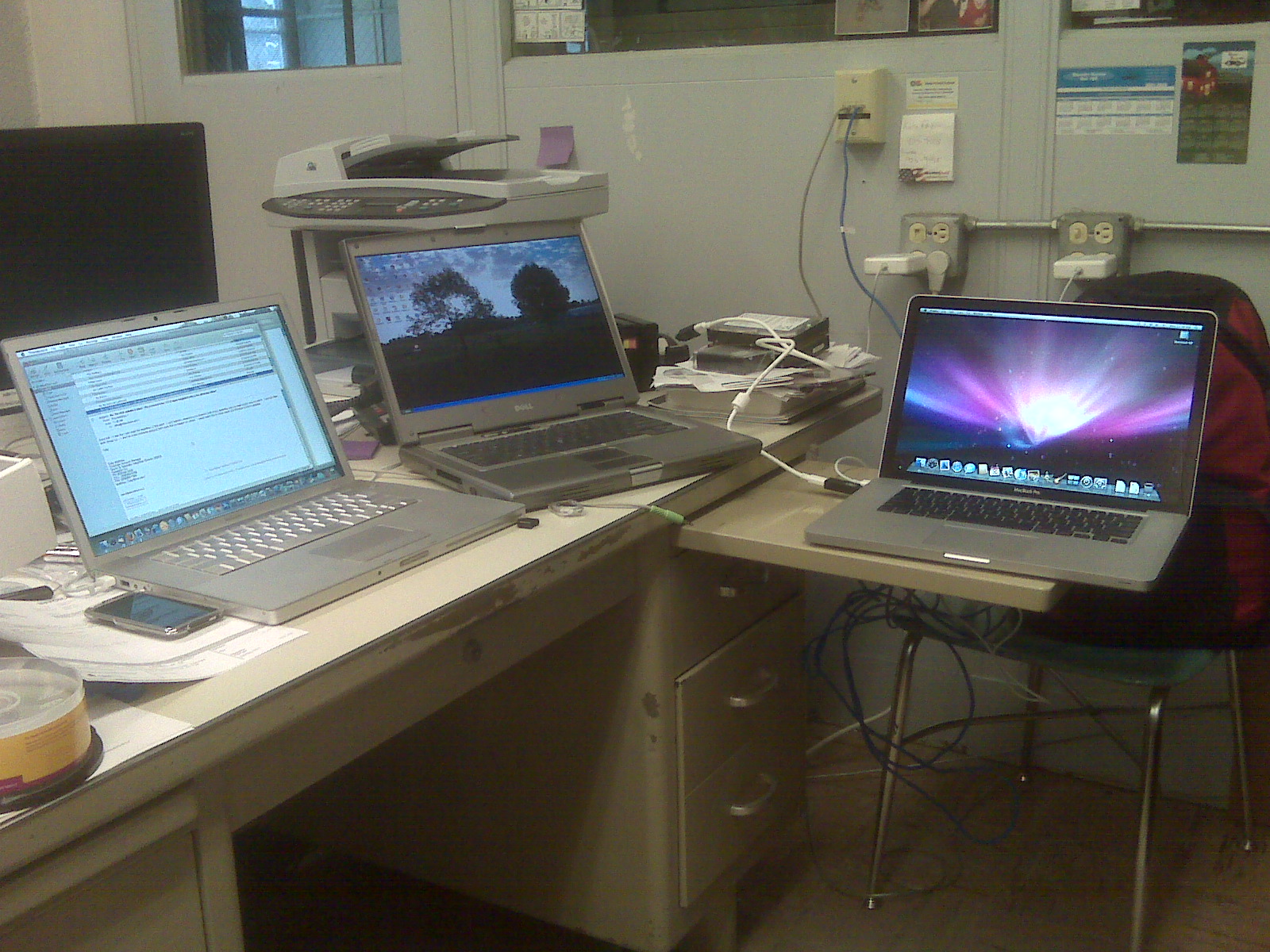This is a photograph of an office desk, likely within a cubicle or a home office setup. Dominating the desk are three open laptops: two appear to be Apple MacBooks, and the third looks like a larger Dell laptop. The desks seem to be a mixture of metal and possibly enamel-painted wood with drawers on both sides and a slide-out tray on the right, holding one of the laptops. The laptops display various screens—one shows an email, another a screensaver, and the third a home screen.

The desk surface is cluttered with numerous items: papers, a BlackBerry cell phone positioned next to the leftmost MacBook, a small stack of blank CDs in a crystal case at the far left, and external hard drives connected to the laptops with tangled cables. There’s also a precariously placed printer or scanner teetering on the edge of the desk, possibly on top of another laptop. Behind the desk, the wall features multiple electrical outlets with various devices plugged in, including chargers for the laptops.

The environment appears utilitarian, with gray walls and possibly windows or a cubicle partition in the background. The setting is dimly lit and somewhat blurry, giving an impression of a busily used and perhaps slightly neglected workspace.